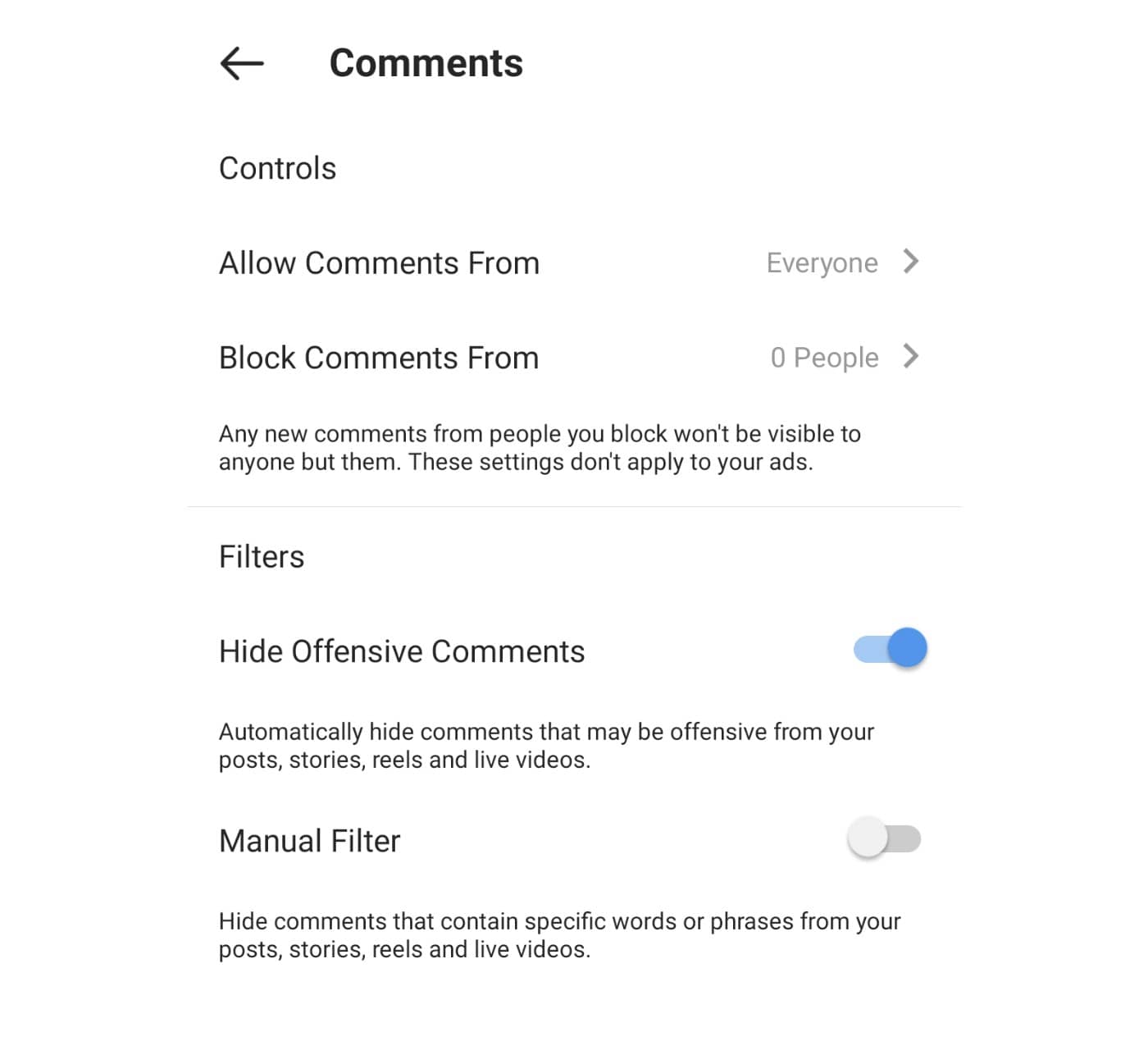Screenshot of a smartphone or other device, featuring a user interface on a white background with blue and black text. In the top left corner, a left-facing arrow indicates the option to go back. Next to it, bold blue text reads "Comments." 

Below the header, in black text, the section labeled "Controls" displays options including "Allow comments from everyone" and "Block comments from 0 people." A note informs that any new comments from blocked individuals will be visible only to them, and these settings do not apply to advertisements. 

A faint gray line separates this section from the next one labeled "Filters." Here, the option to "Hide Offensive Comments" is toggled on, highlighted in blue. Additional text explains that this setting will automatically conceal comments deemed offensive across posts, stories, reels, and live videos.

Another setting, "Manual Filter," is toggled off. This feature allows users to hide comments containing specific words or phrases from their posts, stories, reels, and live videos, though it is currently not enabled.